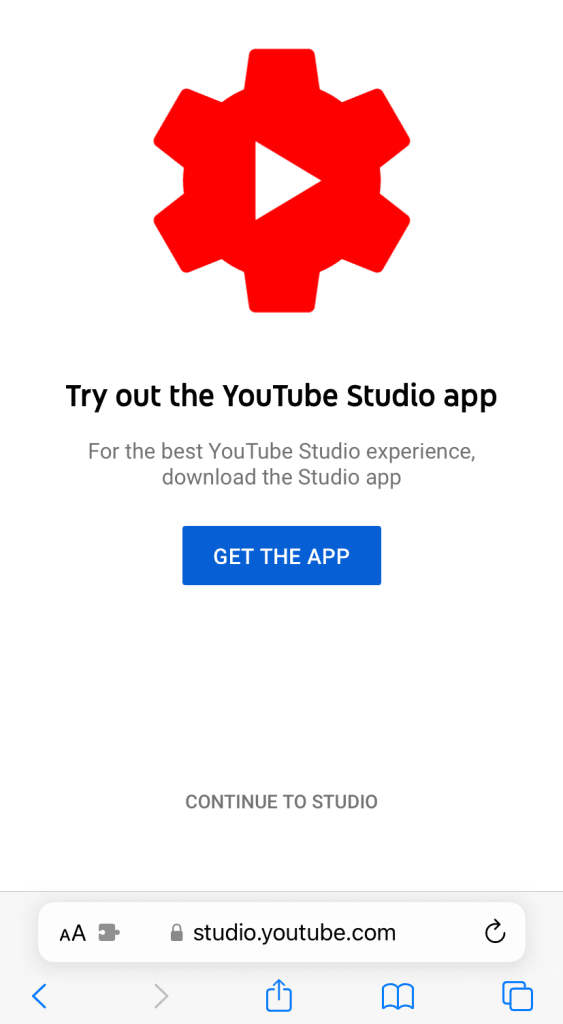The image depicts a screenshot of a web page likely taken from a tablet or a smartphone. The focal point of the web page is a prominent red gear situated at the center, within which lies a white triangle. Directly beneath this graphical element, in bold black text, is the instruction: "Try out the YouTube Studio app." Below this, in regular black text, it reads, "For the best YouTube Studio experience," followed by a new line stating, "Download the Studio app."

A noticeable gap separates this text from a dark blue rectangular button, prominently placed, with "Get the app" written in white in the center. Toward the bottom of the screen, another clickable option appears: "Continue to Studio."

Surrounding the web content is a light gray bezel. Within this bezel, a white rectangle with rounded corners houses the URL and security information. The URL bar starts on the left with two "A" icons (one small and one medium-sized), followed by a puzzle piece, and a lock icon. The URL displayed reads, "studio.youtube.com." On the right-hand side of the URL bar is a refresh icon shaped like a curling arrow pointing to the right.